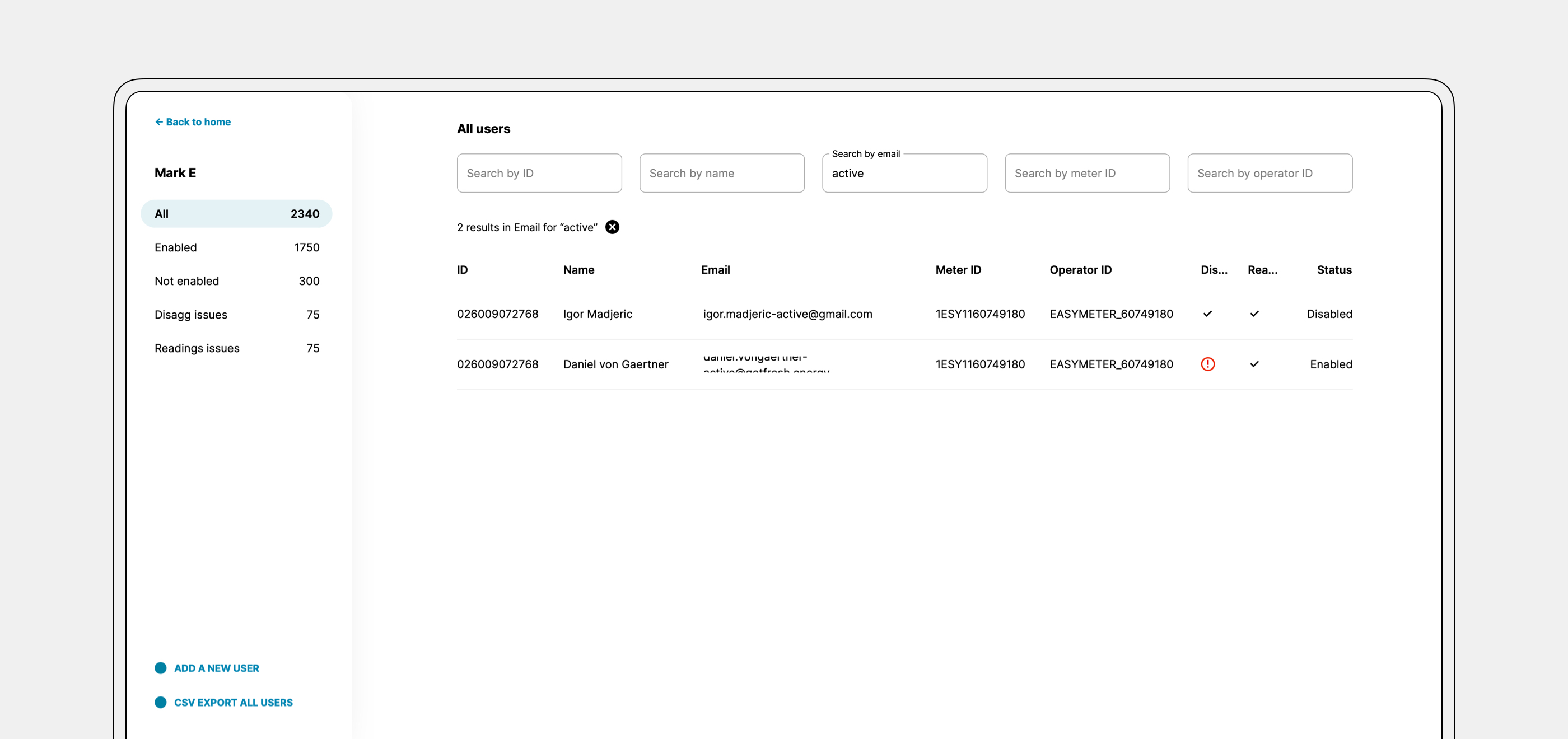The image is a horizontally rectangular representation of a web page displayed on a computer monitor. The frame of the laptop monitor is visible, though the bottom portion is cut off, preventing a full view of the device. The background of the web page is stark white, providing a clean and uncluttered look.

In the top left corner, there is a blue hyperlink labeled "Back to Home." Directly below this, the name "Mark E" is displayed, followed by a vertical list of items. Although the font is very small and some words are not entirely legible, we can make out several key terms. The list includes:

- All (with a number 2340)
- Enabled (with a number 1750)
- Not Enabled (with a number 300)
- DIAG issues (though the exact word "DIAG" is unclear, possibly an abbreviation)
- Issue 75
- Reading issues 75

At the very bottom of this column, there are additional blue hyperlinks: "Add a New User" and "CSV Report Export All Users."

The remaining right side of the page is dominated by various search functionalities. These include:
- All Users
- Search by ID
- Search by Name
- Search by Email (indicated as active)
- Search by Meter ID
- Search by Operator ID

Beneath these search windows, a populated list of search results can be seen. This layout suggests a user interface designed for managing and searching through various user or item records efficiently.